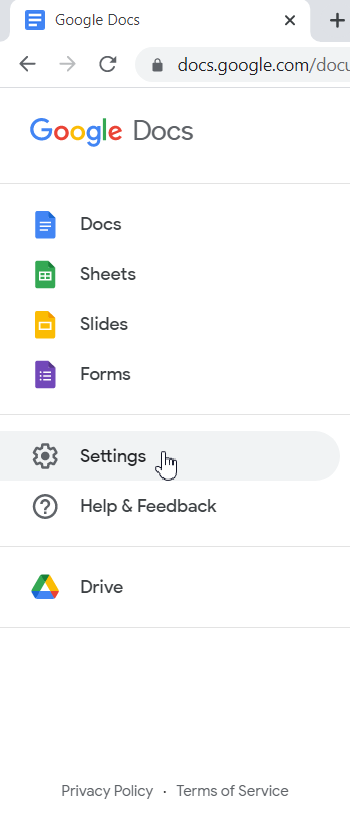A screenshot shows the Google Docs interface open, presumably on a mobile device or tablet. The layout slightly deviates from its typical browser appearance. In the upper left corner, a blue square containing white lines represents the Google Docs icon. Adjacent to the icon, the text "Google Docs" appears in gray. In the upper right corner, a small "X" suggests this is part of an opened tab, and a "+" sign nearby indicates the option to open a new tab.

Directly below, navigation arrows for moving left and right, a refresh button, and a secure lock icon accompany the URL starting with "docs.google.com/docs," which is truncated. The top section of the interface features a white background with gray dividing lines delineating various headings. The first gray line displays "Google Docs" followed by a horizontal list including "Docs," "Sheets," "Slides," and "Forms."

Further down, another gray line contains the word "Settings," highlighted in gray to note the current selection. To the right, a question mark enclosed in a circle, outlined in black, provides access to "Help and Feedback." Just beneath, a line divides sections, featuring a multicolored triangular Drive icon with the label "Drive" next to it. The focal point, a hand-pointing cursor, hovers beside the "Settings" option.